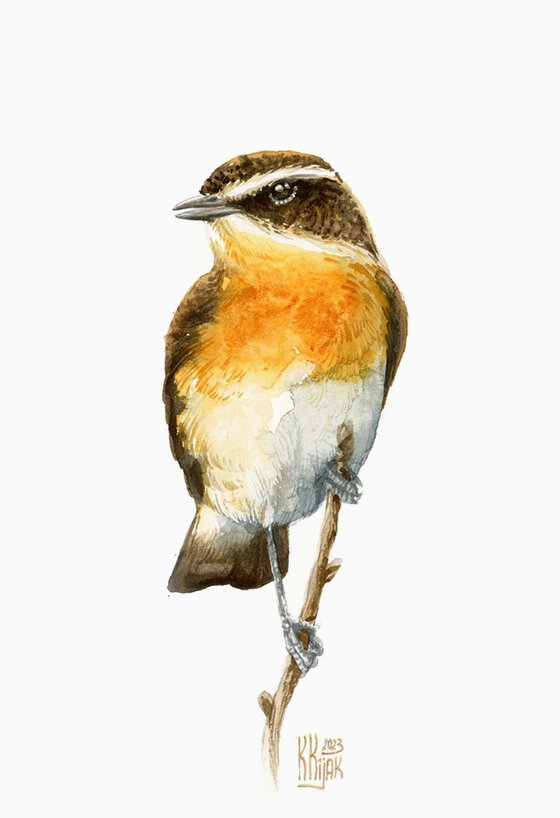This detailed watercolor painting depicts a petite bird, possibly an Oriole, perched gracefully on a lone, brown twig. Its dark wings, brown tail, and white lower body create a striking contrast with its bright orange neck and chest. The head of the bird is particularly intricate, featuring a gray crown and a white stripe running over its fairly large eyes that are accentuated by darker hues with white highlights. The beak is delicate and dark gray-black in color, adding to the bird’s charming appearance. The backdrop is completely white, making the vibrant details of the bird and the twig stand out prominently. The bird’s pose is captured thoughtfully, with one leg perched securely on the branch and the other stretching downward. Notably, the artwork is signed by the artist, potentially named Kijak, with the year 2023 marked in light brown near the bottom center of the piece.